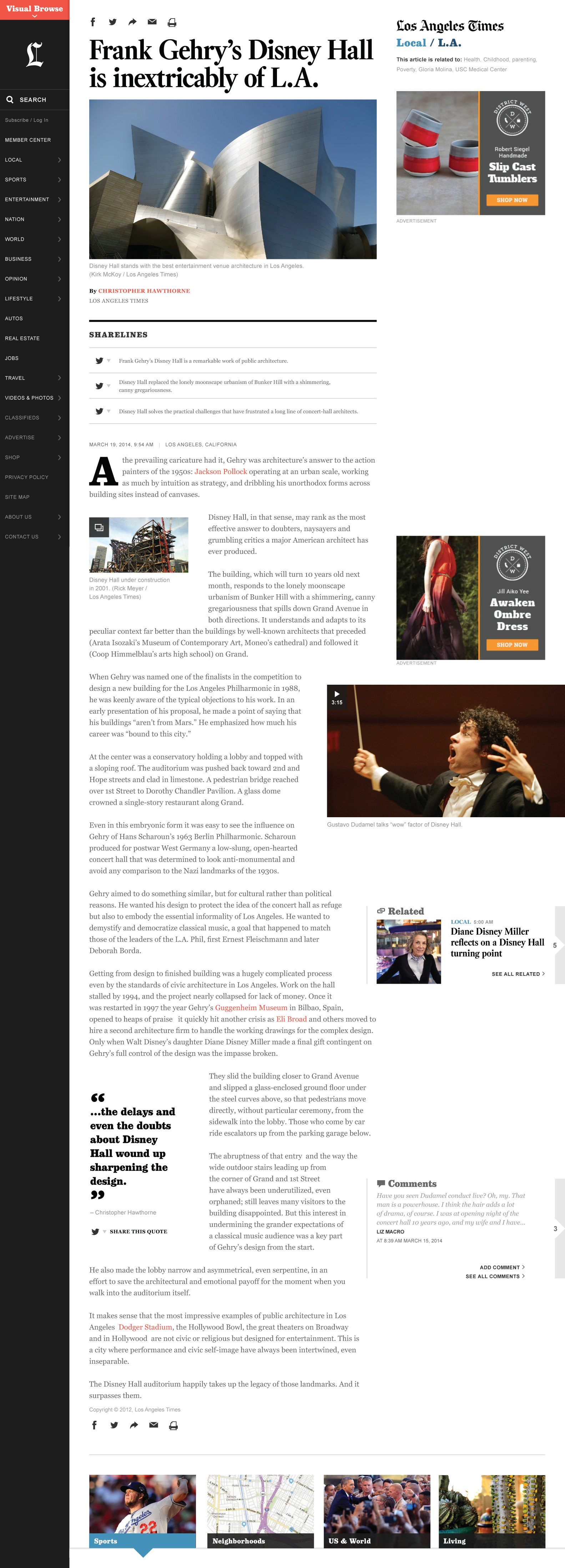A cell phone screenshot captures a detailed feature from the Los Angeles Times, showcasing Frank Gehry's iconic Disney Hall. The top of the image prominently displays the caption: "Frank Gehry's Disney Hall is inextricably linked to LA," accompanied by a high-resolution photograph of the building's striking geometric design. Below the image, another caption reads, "Disney Hall stands with the best entertainment venue architecture in Los Angeles," credited to writer Christopher Hawthorne. 

The article, dated March 19, 2014, at 9:54 AM in Los Angeles, California, continues below, enriched with share buttons for social media platforms such as Twitter. The piece includes several historic and construction-related images, offering a visual journey through the development of the hall. One photo, dated 2001, shows Disney Hall under construction, while another features a conductor named Gavesto Damali discussing the 'Wow Factor' of the venue. The article, comprehensive in scope, visually stretches throughout the length of the cell phone screenshot, providing an in-depth look at one of Los Angeles's architectural gems.